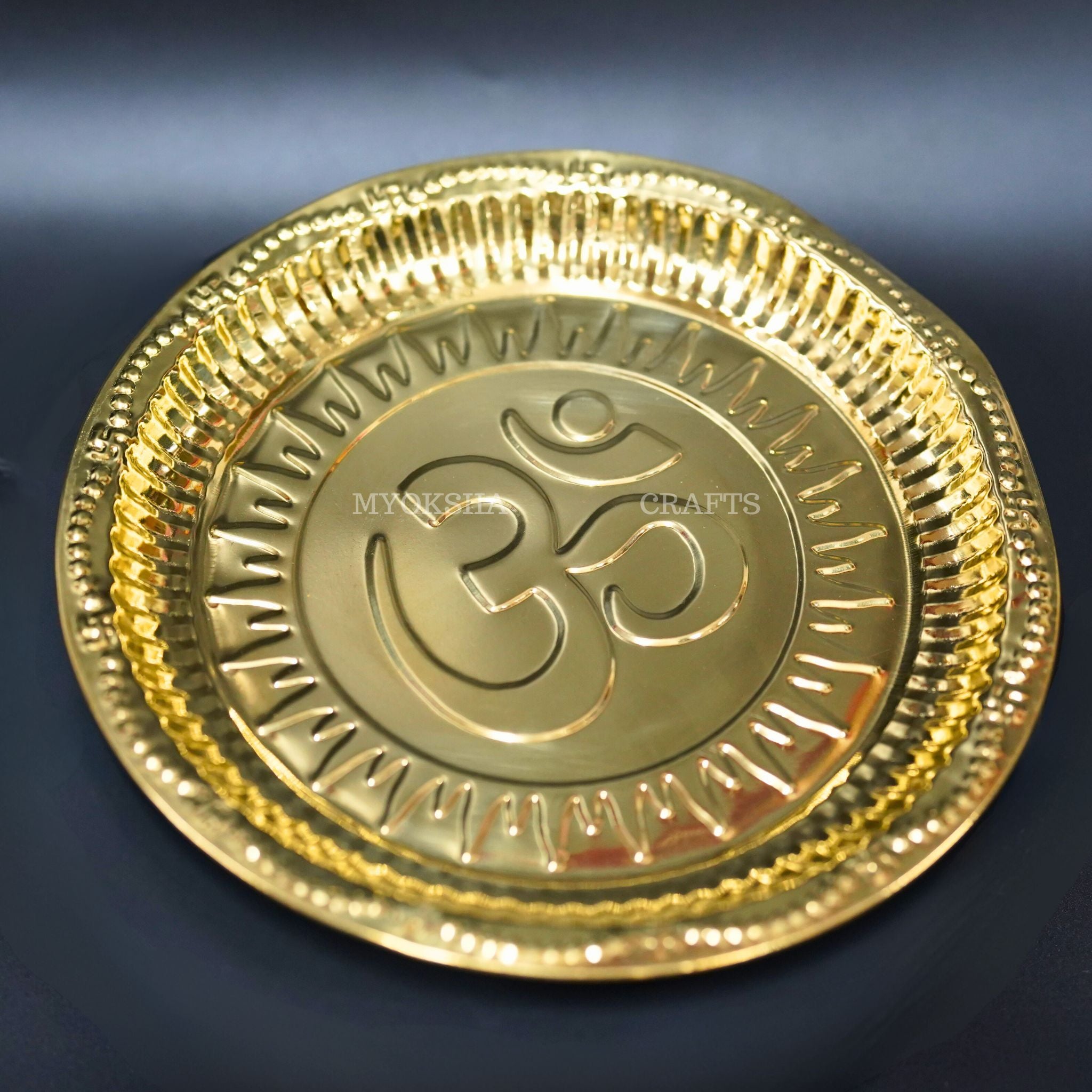The image features a meticulously crafted, circular gold dish, potentially an ashtray, prominently displaying intricate details. At its center is the symbol associated with Namaste or Aum, featuring a large number three with a small circle and line beneath it and a tail resembling a backwards C, suggesting it might be in a different language. The design is surrounded by imprints resembling molars, adding to the ornate craftsmanship. The rim around these details is a brighter gold, enhancing the dish's visual appeal. The background is a gradient of grey and white, showcasing the dish with a sun motif and extending rays at the bottom. The name "Myoksha Crafts" is prominently watermarked towards the center, indicating the craftsmanship and possibly hinting at a commercial or artistic advertisement. Despite being perceived as a "fake" gold item, the level of detail suggests intricate, possibly 3D-printed design on a blue and white backdrop.